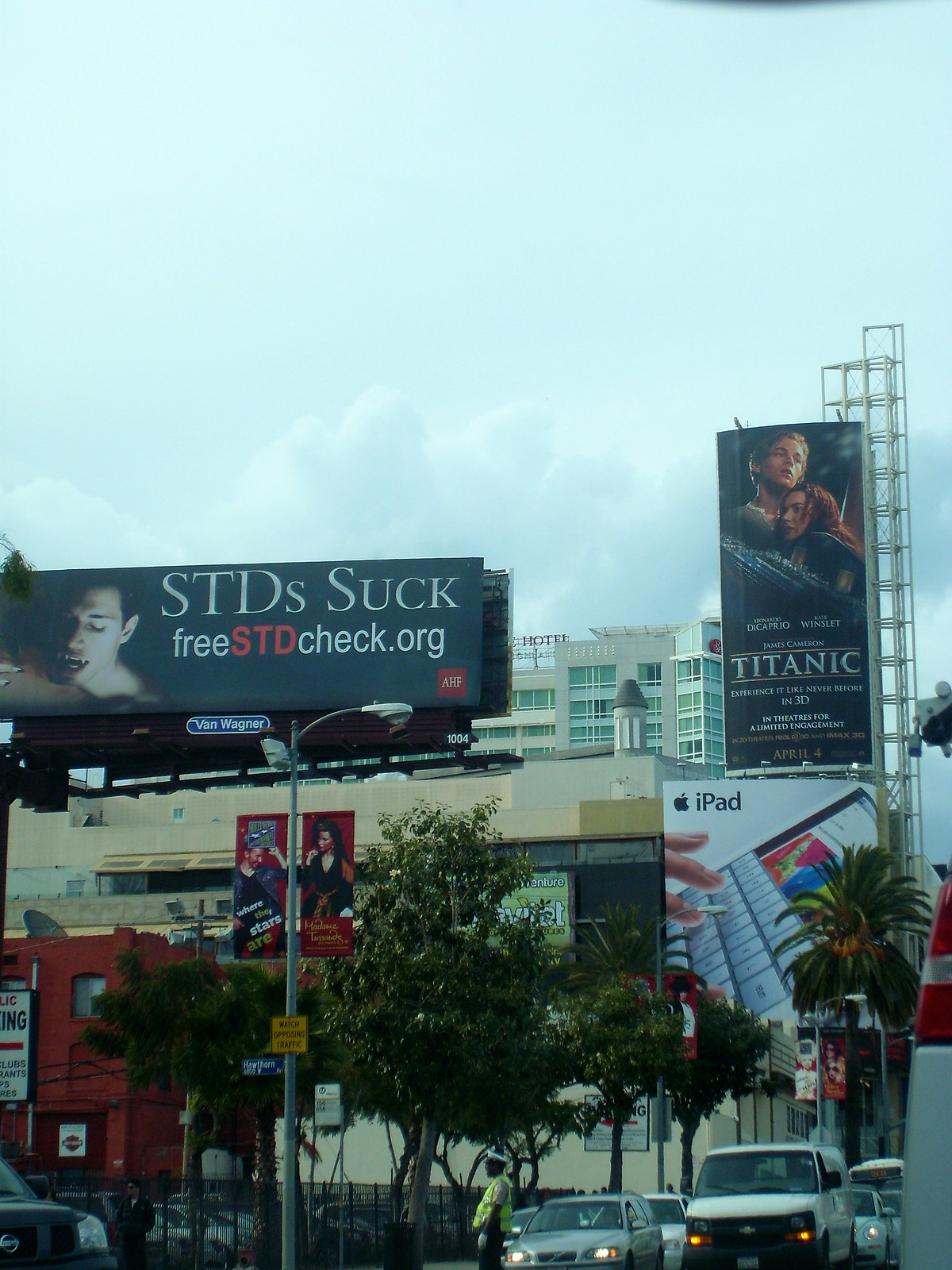The image captures a lively urban streetscape bustling with activity. At the forefront, several cars are neatly lined up, with a person donning a green vest standing in front of them, possibly directing traffic or serving in a supervisory role. Toward the middle-left section of the frame, there’s a prominently positioned light post adorned with a yellow sign, which slightly breaks the symmetry but adds to the scene’s realism.

In the background, a variety of buildings stretch upwards, their facades interspersed with vibrant advertisements that vie for attention. Among these, three signs particularly stand out. On the left, a bold sign reads "STD Suck: freeSTDcheck.org," serving as a public health announcement. To the right, an eye-catching Titanic-themed advertisement features a dramatic image of a man, a woman, and a ship. Centered and elevated, a clean, white sign announces the iPad with a sleek image of the tablet.

The sky overhead is a gentle light blue, decorated with sporadic clouds, providing a serene contrast to the dynamic street scene below. Every element in the frame—from the tall buildings with their unique ads to the person in the green vest—contributes to the rich tapestry of city life depicted in the photograph.